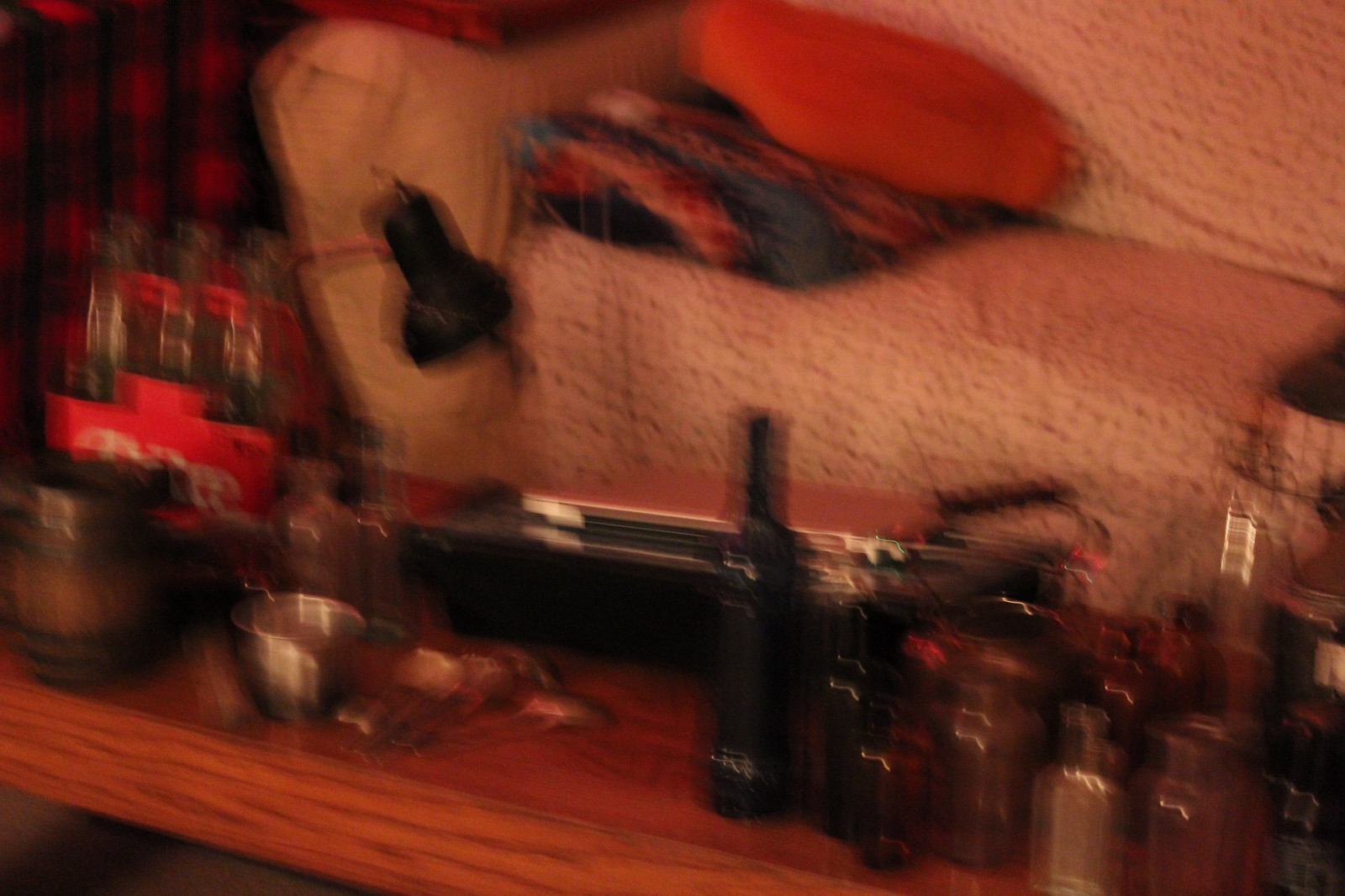The image presented is a photograph, wider than it is tall, capturing the interior of a cozy yet cluttered living space. The scene is hazy with a soft blur, giving it a nostalgic, almost dreamlike quality. Central to the composition is a coffee table crowded with a variety of items: a box containing Coca-Cola glass bottles, several measuring cups, and a collection of various bottles in the lower right-hand corner. 

Behind the table, a sofa spans from the center of the image to the upper right corner. The sofa is draped with a patterned blanket, adding a touch of color and texture to the setting. On the left side of the sofa, there is another folded blanket with an orange pillow placed neatly on top.

To the left on the coffee table, a small desk lamp stands, casting a gentle glow over the nearest objects. In the upper left corner above the sofa, there is a blurred mix of black and red patterns that might be another blanket or a different fabric, adding an additional layer of intrigue and warmth to the scene. The overall ambiance of the image is that of a lived-in, homely space brimming with everyday life and comfort.